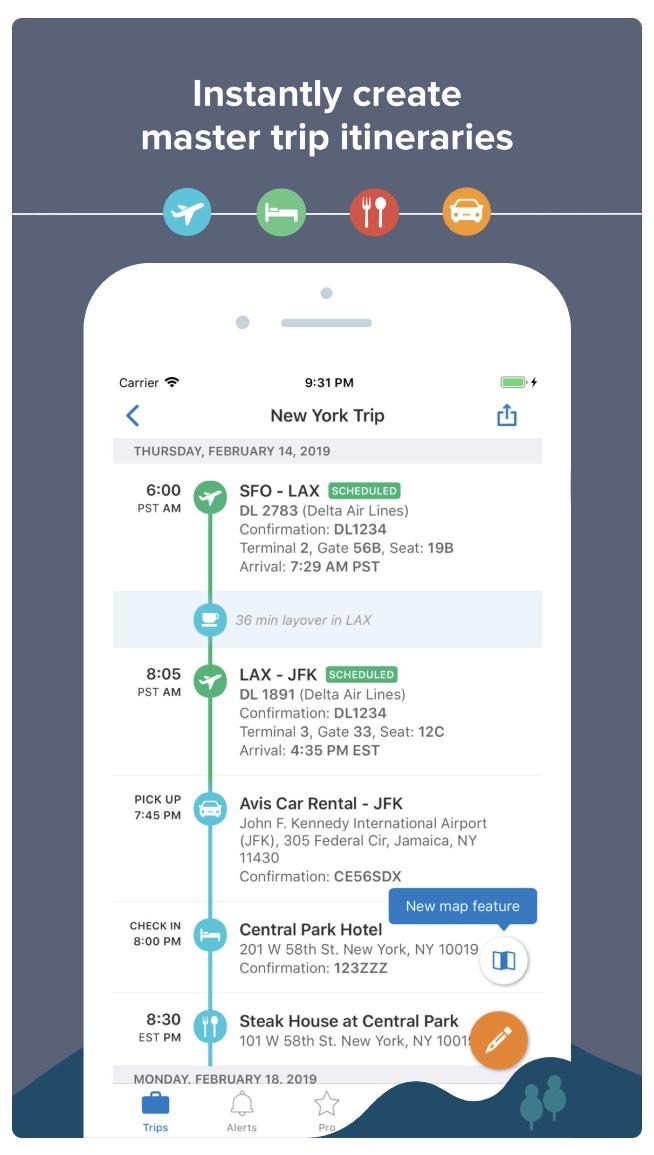The screenshot displayed on a smartphone shows a detailed Master Trip itinerary interface against a green backdrop. At the top of the screen, there are icons representing different travel categories: an airplane taking off, a bed for accommodations, dining utensils (fork and spoon), and a car for auto rentals. The current screen displays a planned trip to New York, with the device's time noted as 9:31 p.m. In the top left corner, there is a carrier signal indicator, and in the top right corner, the battery is shown to be fully charged. 

The itinerary details include the travel date: Thursday, February 14th, 2019, and the journey starting at 6:00 a.m. Pacific Standard Time with a flight from SFO to LAX. The information section outlines the flight's timing, terminals, and confirmation details. Following this, there is a 36-minute layover at LAX, departing at 8:05 a.m. PST with a scheduled flight from LAX to JFK. 

Additional itinerary elements include a coffee cup icon representing a brief layover and necessary flight information, such as confirmation codes and arrival terminals. Upon arrival at JFK, there is a planned car rental pickup from Avis at 7:45 p.m., with further confirmation details provided.

The itinerary continues with hotel check-in details at Central Park Hotel, located at 201 West 58th Street, New York, including confirmation numbers. Dining reservations are also noted, with a meal planned at a steakhouse on the same street (101 West 58th Street) on Monday, February 18th, 2019.

The screen's bottom portion is mostly cut off, but visible content includes navigation buttons and avatars labeled “trips,” “alerts,” and “pro.” Lastly, the screen background fades to dark blue, indicating a transition in the interface.